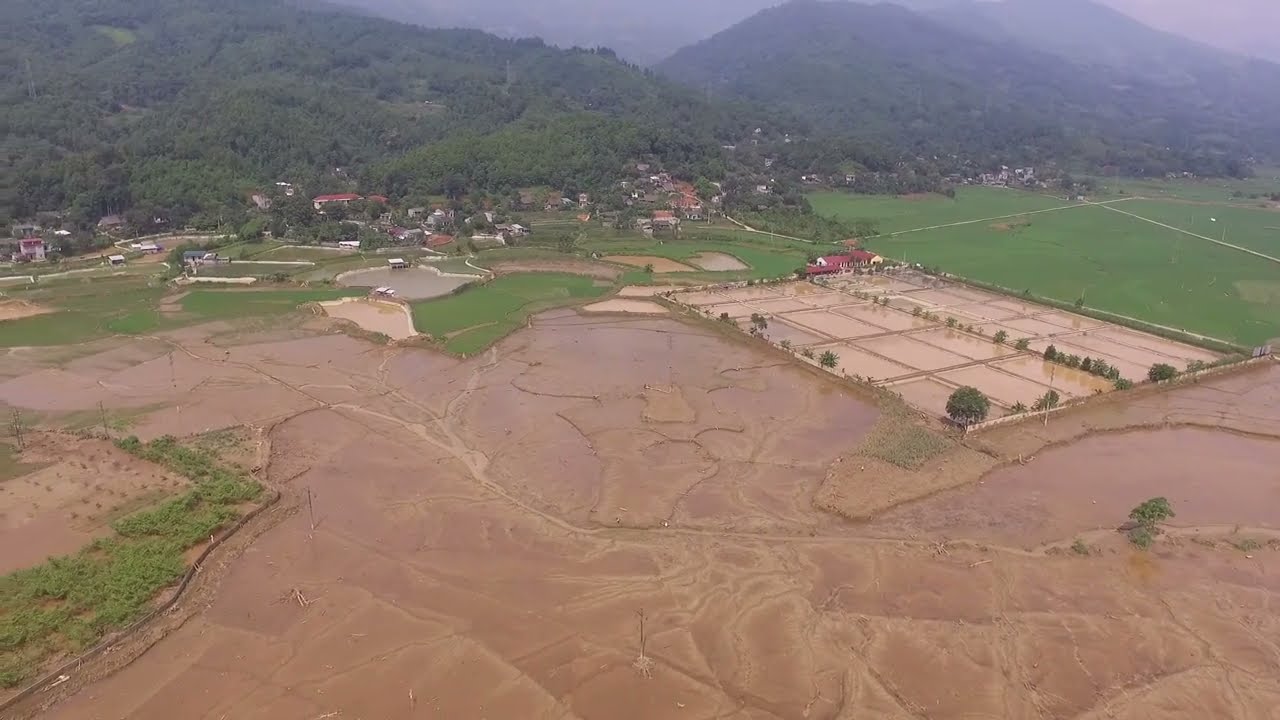In this highly detailed aerial landscape photograph, green rolling hills or mountains span the upper part of the image, adorned with lush forests and vegetation. Below these verdant peaks lie numerous small homes, their rooftops ranging in color from red and white to shades of orange and tan, dotting the middle ground. In the central right portion, a notable white house with a red roof is positioned amidst rectangular, flooded fields that resemble rice paddies, distinguished by a waterlogged brown expanse surrounding them. The foreground presents a contrasting scene of vast muddy plains and possibly recently flooded areas, interspersed with patches of green grass at the base of the hills and along the left edge of the photograph. Gray or white cement pathways meander through the landscape, adding to the sense of an organized, yet rural environment. The distant background contains a light fog, giving a hazy touch to this extensive, richly textured, and vibrant outdoor view from a high vantage point.